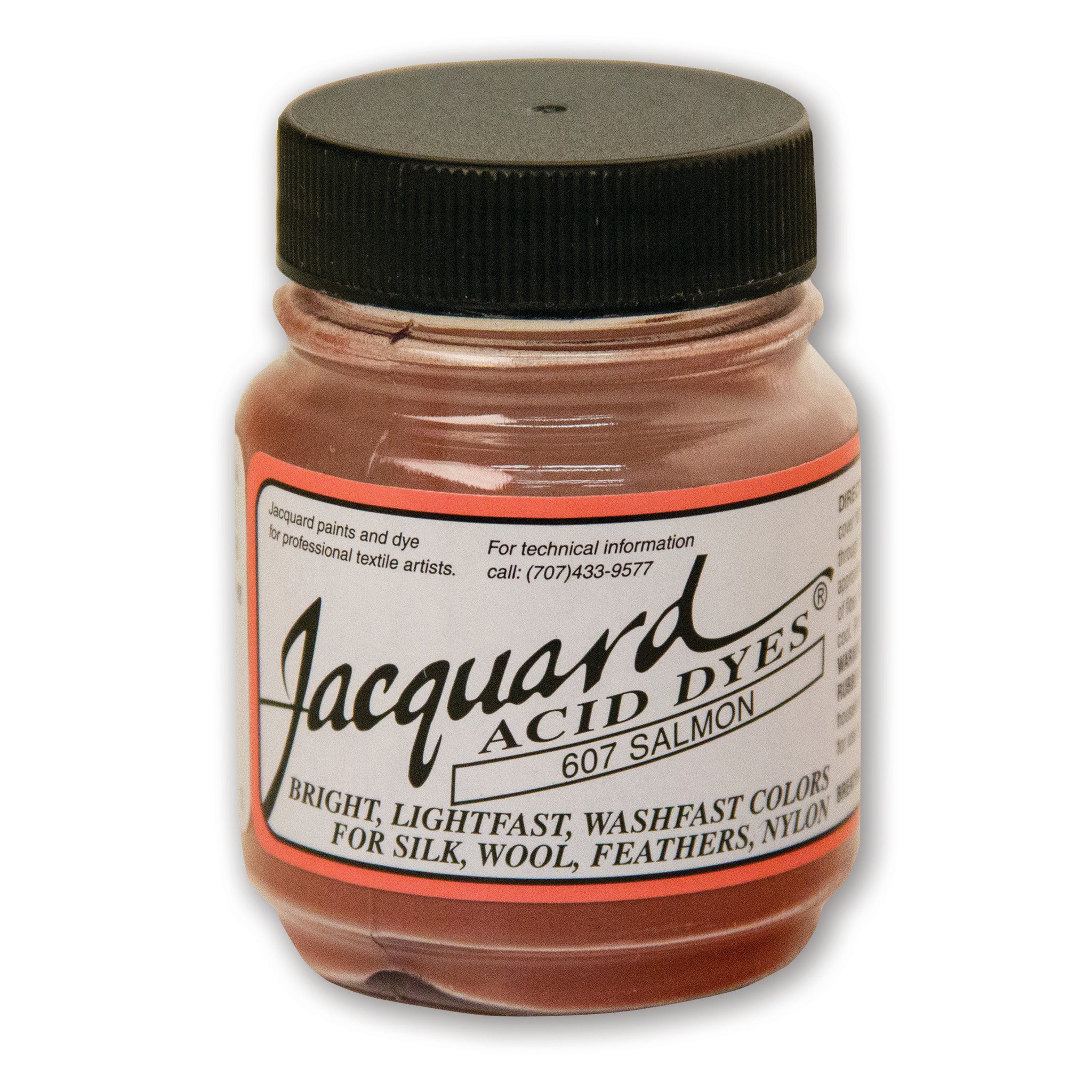The image depicts a small glass bottle of Jacquard Acid Dyes, specifically the 607 Salmon color. The bottle is about the size of a nail polish bottle, roughly five to six inches tall. It features a black twist cap and contains a substance that appears to be a reddish-brown or auburn color, almost resembling sand. The bottle's label has a salmon-colored border with a white background. Prominently displayed at the top in large black cursive font is the brand name "Jacquard," with "Acid Dyes" written below it in non-cursive font. Within a rectangle on the label, the color code "607 Salmon" is indicated. Additional text at the bottom of the label highlights that the dyes offer bright, lightfast, and washfast colors suitable for silk, wool, feathers, and nylon. The left side of the label includes a description stating "Jacquard paints and dye for professional textile artists," and there's a phone number provided for technical information at the top. The bottle is photographed against a white background, clearly showcasing its details.